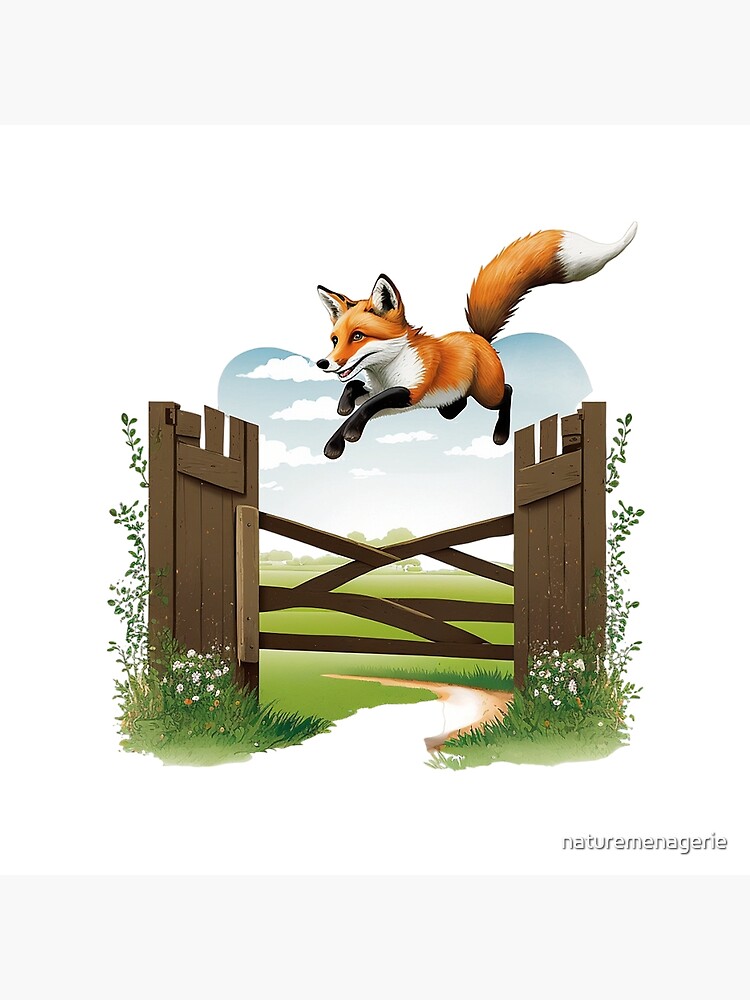The image depicts a colorful, hand-drawn artwork reminiscent of a children's book illustration. In the center, two brown wooden fence posts support a small gate, which is surrounded by patches of grass, white flowers, and a vine climbing up the sides. A vibrant cartoonish fox, primarily colored in orange with a white belly, muzzle, chest, tail tip, and ear highlights, is depicted mid-air as it leaps over the gate. The fox has black legs and features an oddly extra set of legs, giving it an unnatural appearance, likely indicating the image was AI-generated. Below the gate runs a stream with muddy water, and in the distance, trees, a blue sky, and clouds that seem to form a heart shape add to the whimsical scene.